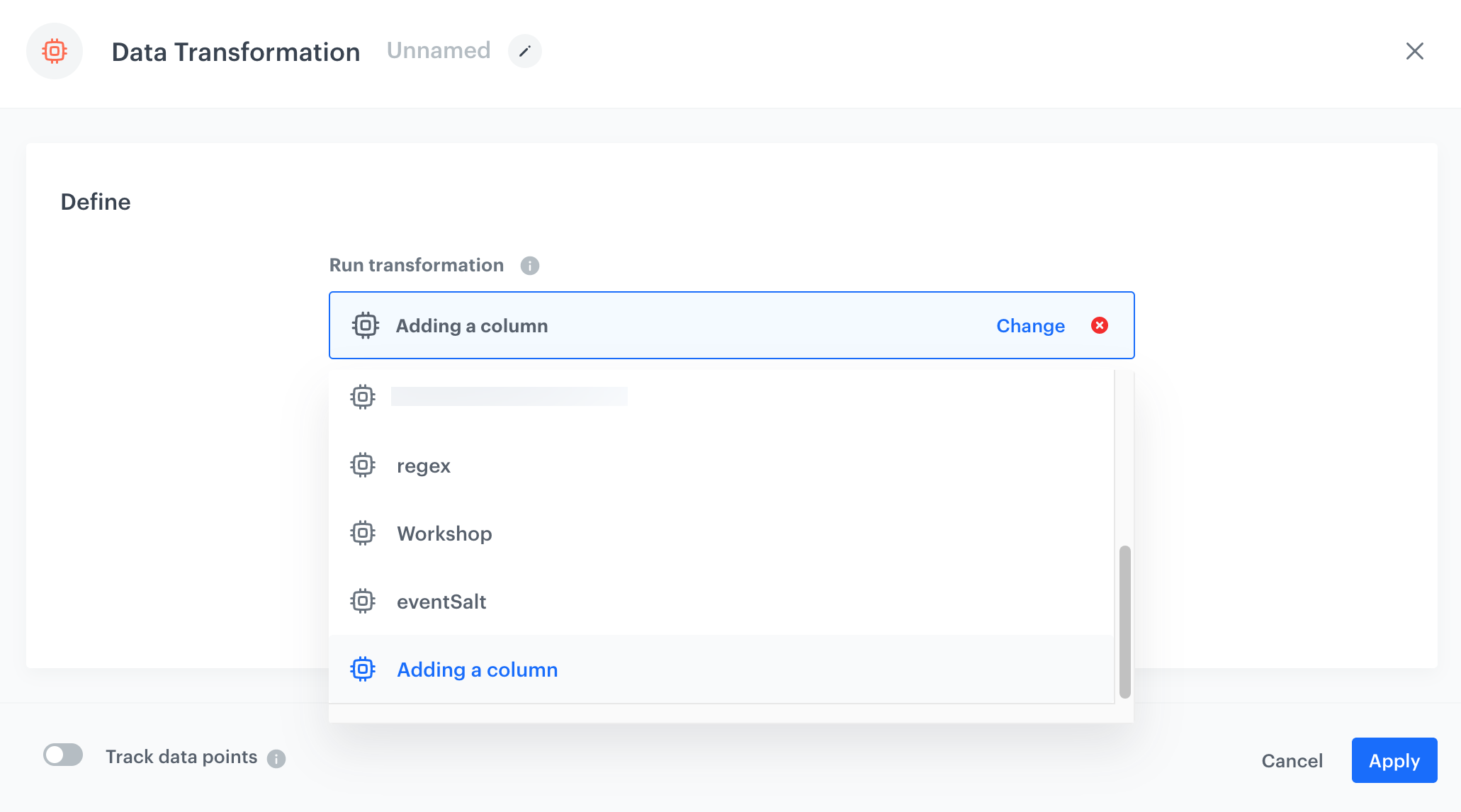Here's a detailed and cleaned-up caption for the image:

---

The screenshot showcases a website interface with a minimalist all-white background. At the top left corner of the screen, there is a small circular icon featuring a red button inside, resembling a target. To its immediate right, the bold text reads "Data Transformation," followed by the grayed-out word "Unnamed" alongside a small edit icon. Towards the far right, there is a standard "X" button used for closing the window.

Below this top bar, a light gray border encloses another white section. At the top left of this section, the word "Define" is displayed. In the middle, there is a white text box containing the phrase "Run Transformation" accompanied by an informational "i" button.

Further down, a list of options in a blueish tone begins with "Adding Column," which is highlighted. To the right of this option, there is a red "X" button labeled "Change." Below the highlighted option, a sequence of unselected options includes "Blank," "Regex," "Workshop," "Salt," and once more, "Adding Column."

Just beneath this list, within the light gray border, there is a toggleable option labeled "Track Data Points," with an informational "i" button indicating it is currently turned off. To the far right, there are "Cancel" and "Apply" buttons, respectively.